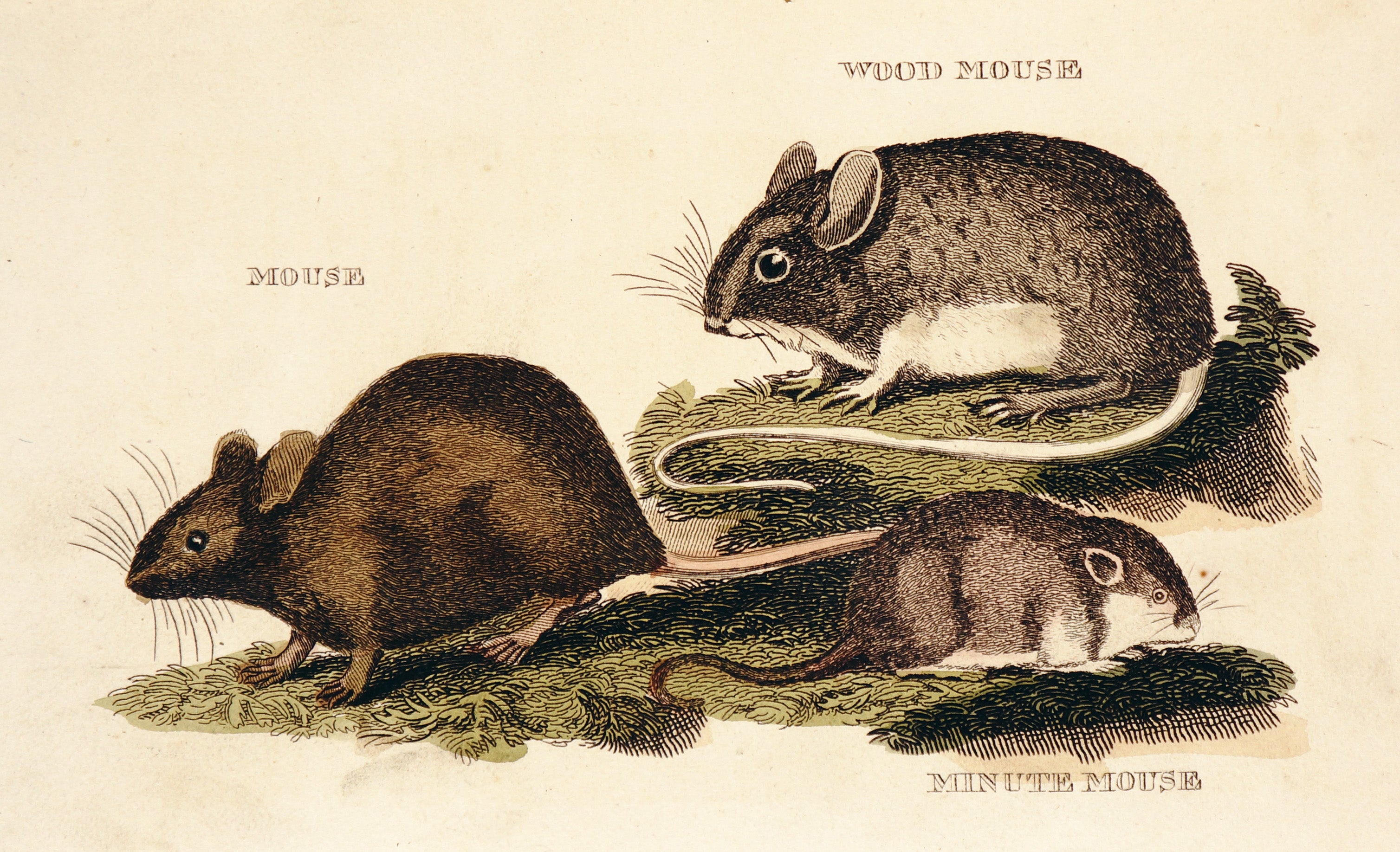This image is a vintage-style drawing on tan parchment, reminiscent of a biology or woodland field manual, depicting three distinct types of mice with faded colors primarily in shades of black, brown, white, and a touch of green. On the left, a larger, darker mouse labeled simply "mouse" is sitting on a patch of grass, with prominent whiskers, ears, and a robust body. Above and to the right of it is a "wood mouse," lighter in color, with a white underbelly, chin, and throat, looking off to the left. At the bottom right, the smallest mouse, called "minute mouse," has a brownish-gray coat, a dark tail, and white markings on its belly, legs, cheeks, throat, and parts of its face, gazing to the right. All mice appear to be hand-drawn with intricate detail, enhancing the vintage and educational feel of the artwork.